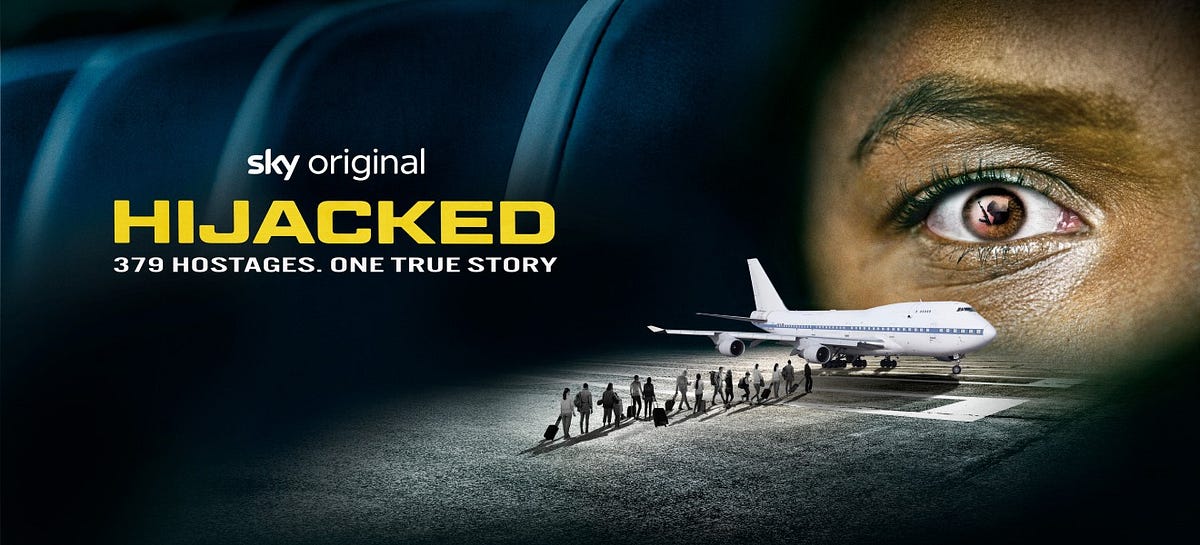This image serves as an advertisement for a movie titled "Hijacked," produced as a Sky Original. It features a dark blue, almost black background with mysterious and foreboding elements. The layout is rectangular and significantly wider than it is tall. 

On the left side of the image, slightly towards the top, the words "Sky Original" are written in bold, lowercase white letters, representing the Sky Network's branding. Below this, the title "HIJACKED" stands out in large, bold yellow all-caps text. Directly underneath the title, a tagline in white text reads: "379 hostages. One true story."

On the right side of the poster, occupying the upper right corner is a close-up of a person's right eye. The eye, which is wide open and has a brown iris, appears to be from a person with slightly brown skin, suggesting a sense of panic or urgency. Reflected in the eye is the startling image of a man holding a rifle, adding to the tension and ominous tone of the poster.

Beneath the eye and slightly towards the lower center, there's a smaller image of a white airplane positioned on a runway. Near the airplane, a line of passengers with luggage is depicted, suggesting they are about to board. The passengers and the plane aren't proportionally accurate, adding to the surreal and dramatic feel of the image. The scene is set against a dark tarmac, enhancing the overall sense of night and mystery.

The upper left corner behind the word "Hijacked" subtly shows blue airplane seats, shrouded in shadow, contributing to the dark and enigmatic atmosphere of the poster.